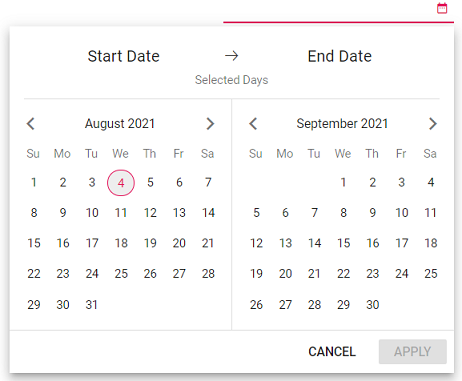The image depicts a calendar interface with a white background, displaying an event timeline from August 2021 to September 2021. The start date, "August 2021," is on the left-hand side, covering the period from Sunday, August 1st to Tuesday, August 31st, with the number 4 distinctly highlighted in red and circled. The end date, "September 2021," is on the right-hand side, showing days from Wednesday, September 1st to Thursday, September 30th. At the top-right corner of the end date section, there's a horizontal purple line extending rightwards with an arrow pointing to the right in its center. Adjacent to this arrow, in the top-right corner of the image, is a calendar icon, a small square with red accents. Below the September calendar, there are two buttons: "Cancel" and "Apply," with "Apply" shaded in gray.